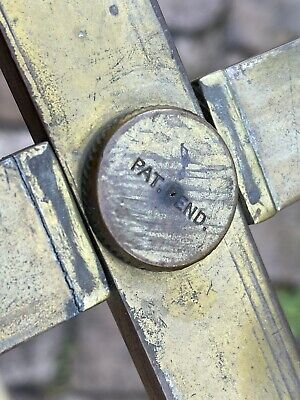This image depicts an aged metal measuring device, predominantly showcasing a cross-shaped structure. The device appears to be gold in color, with significant portions of the paint peeling off, revealing a metal substrate that might be pewter or steel. The intersection of the cross features a circular, ridged knob inscribed with "PAT. PEND." and marked with numerous scratches from prolonged use or deliberate scraping. Each arm of the cross-like device, characterized by noticeable wear and faded surfaces, appears to have square or rectangular end caps, though their method of attachment (welded or screwed) is unclear due to the absence of visible fasteners. The left and right arms of the device seem to be designed for movement or adjustment, potentially sliding past each other. The background is blurred, possibly a stone wall, adding to the worn, utilitarian aesthetic of the device. Overall, the heavily scratched, darkened edges and textured surface highlight the object's age and extensive usage.